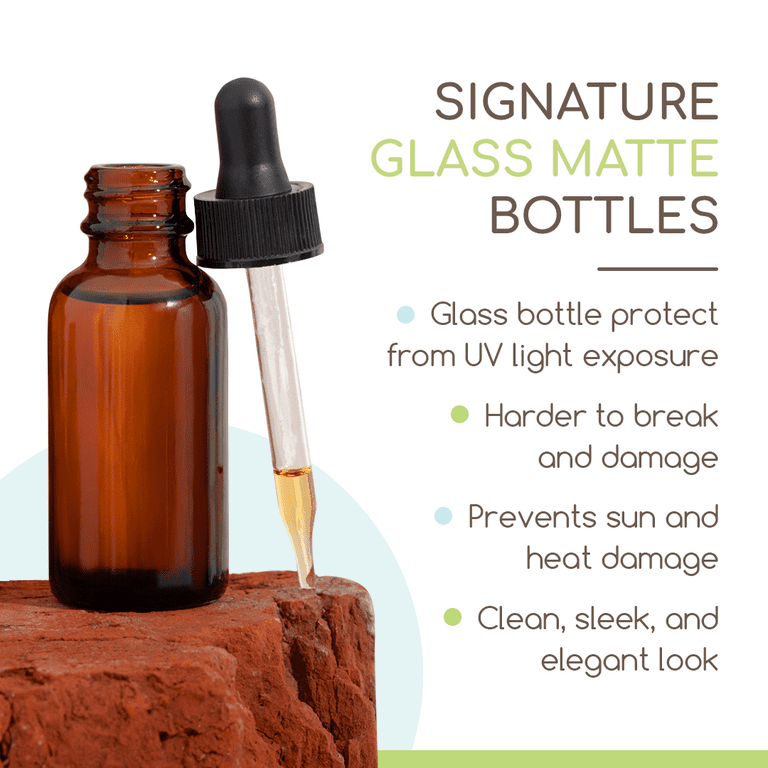The image is a detailed advertisement showcasing a brown dropper bottle filled to the brim with a liquid, likely an oil, and an accompanying dropper placed upright to its right. The dropper contains a yellowish-amber liquid filling about a third of its length. Both the bottle and the dropper rest on a surface resembling a rough, rust-colored rock. In the background, a blue semicircle adds a contrasting element to the composition. To the right, the text "Signature Glass Matte Bottles" is prominently displayed, followed by a horizontal line and a series of bullet points describing the product's features: "Glass bottles protect from UV light exposure," "Hard to break and damage," "Prevent sun and heat damage," and "Clean, sleek, and elegant look." Each bullet point is marked with either a green or blue dot, reinforcing the product's advertised qualities.